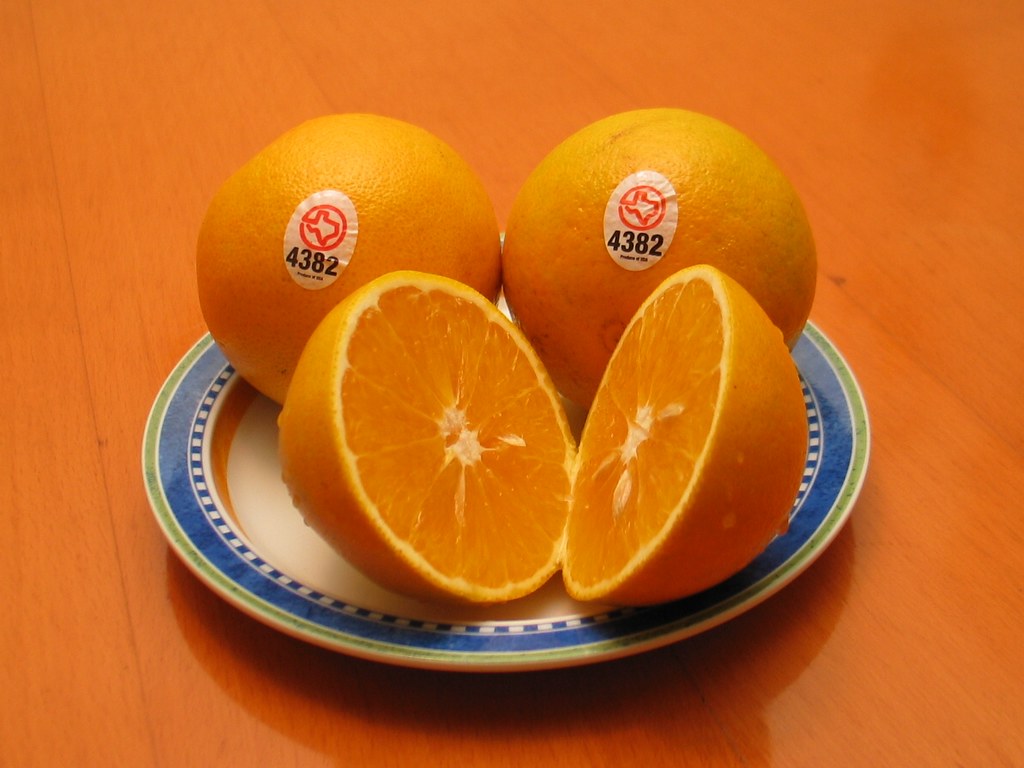This image features three oranges beautifully arranged on a small, round plate with intricate detailing, set against a medium orange-ish wooden table with a shiny, lacquer finish. The plate itself is white-centered with an elaborate trim: starting with an orange border, followed by a blue and white checkered band, and then a solid blue band with an outermost green ring. Two whole oranges, each adorned with a PLU sticker displaying the number 4382 and an outline of the state of Texas, are positioned in the back. One orange, sliced in half to reveal its juicy, seed-filled interior, takes the center stage in the front. The vivid oranges contrast sharply with the plate's intricate rim and the glimmering wooden tabletop, creating a visually appealing and detailed composition.